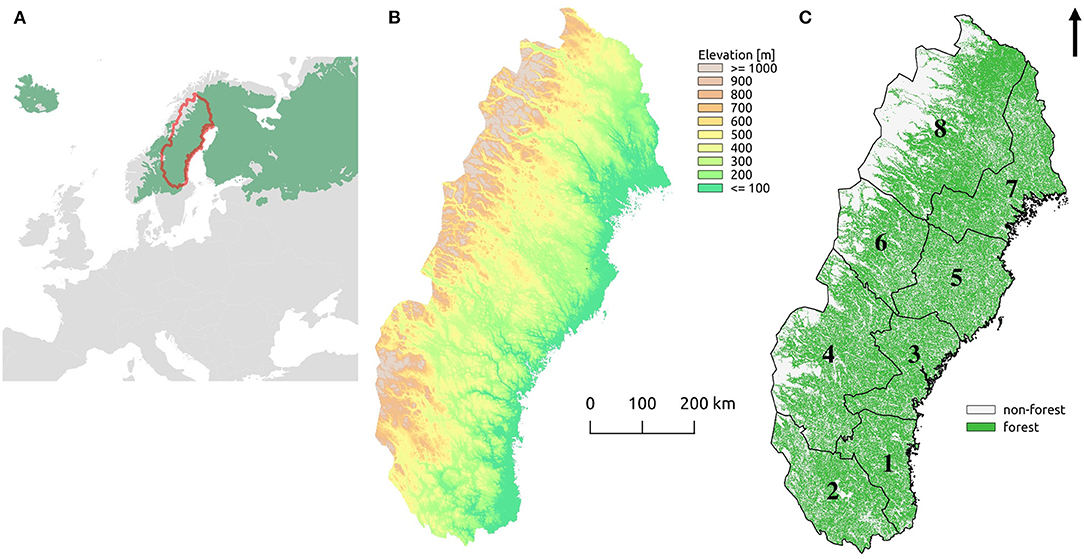The image is a computer-generated topographic collage consisting of three maps labeled A, B, and C, displayed side by side against a white background. 

- **Map A** (left): This section presents a far-off, zoomed-out view of a continent-like landmass divided into two regions colored in green and grey. Notably, a red outline encircles an area of interest at the top of this map, drawing attention for further analysis.

- **Map B** (middle): This map zooms into the region highlighted in Map A, showcasing elevation data through a gradient of colors ranging from light purple, light pink, and light orange to darker shades of green. The accompanying elevation legend on the right side specifies the elevation levels in meters (m), with the higher elevations depicted in greener tones.

- **Map C** (right): This section categorizes the area into forest and non-forest regions, marked respectively in green and white. The map is divided into eight numbered sections, providing detailed segmentation of the land cover.

Each map offers a different layer of information, weaving together a comprehensive topographical and ecological analysis.